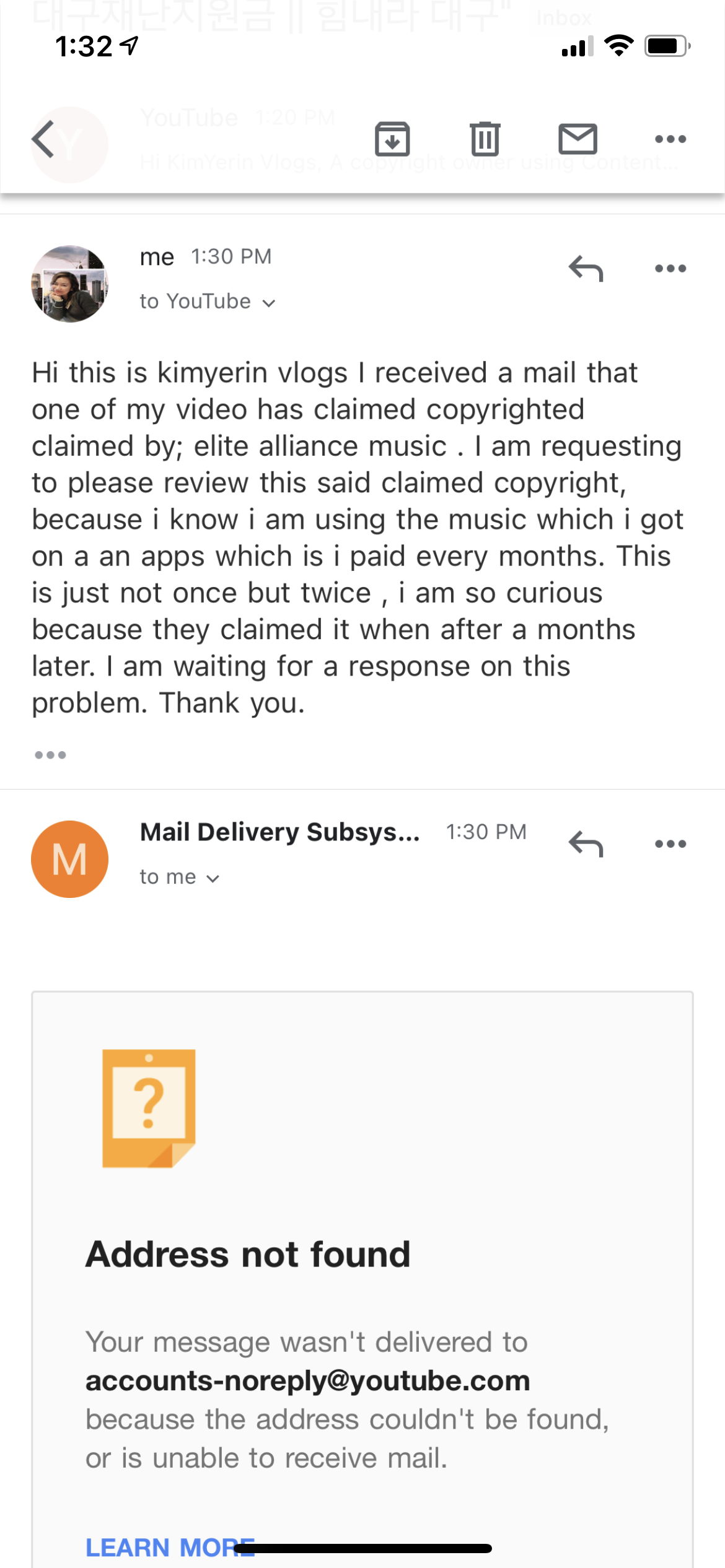This image is a screenshot from the Gmail app, predominantly featuring a white background. At the top right corner, there are icons indicating Wi-Fi connectivity and battery status. The top left corner displays the time, "1:32," in black text.

Beneath the battery percentage icon, there is a dark gray box. Adjacent to this box on the right, there is a gray trash can icon, followed by a gray envelope icon, and three horizontal dots symbolizing more options.

On the far left, there's a gray arrow pointing to the left, indicating the option to navigate back. Below this arrow, there's a profile picture of a girl, accompanied by the black text "me" on the right, indicating that the user is composing an email.

The email body beneath the profile picture reads:
"Hi, this is Kim Yaron Vlogs. I received a mail that one of my video has been claimed copyrighted, claimed by: Elite Alliance Music. I am requesting to please review this said claimed copyright because I know I'm using the music which I got on AN apps, which is I paid every month. This is just not once but twice. I am so curious because they claimed it after months later. I am waiting for a response on this problem. Thank you."

Below this message, there is a reply with the sender's name in bold black text, reading "Mail Delivery Subsystem." To the left of the sender's name is a circular orange profile picture with a white "M" inside. Directly below, there is a light gray box featuring an orange document icon at the top.

Following the icon, the black text reads "Address not found." Underneath, there is light gray text stating, "Your message wasn't delivered to," followed by bold black text, "accounts-no-reply@youtube.com." Continuing, the light gray text explains, "because the address couldn't be found or is unable to receive mail."

At the bottom left of the image, all in caps and in blue text, is the option to "LEARN MORE."